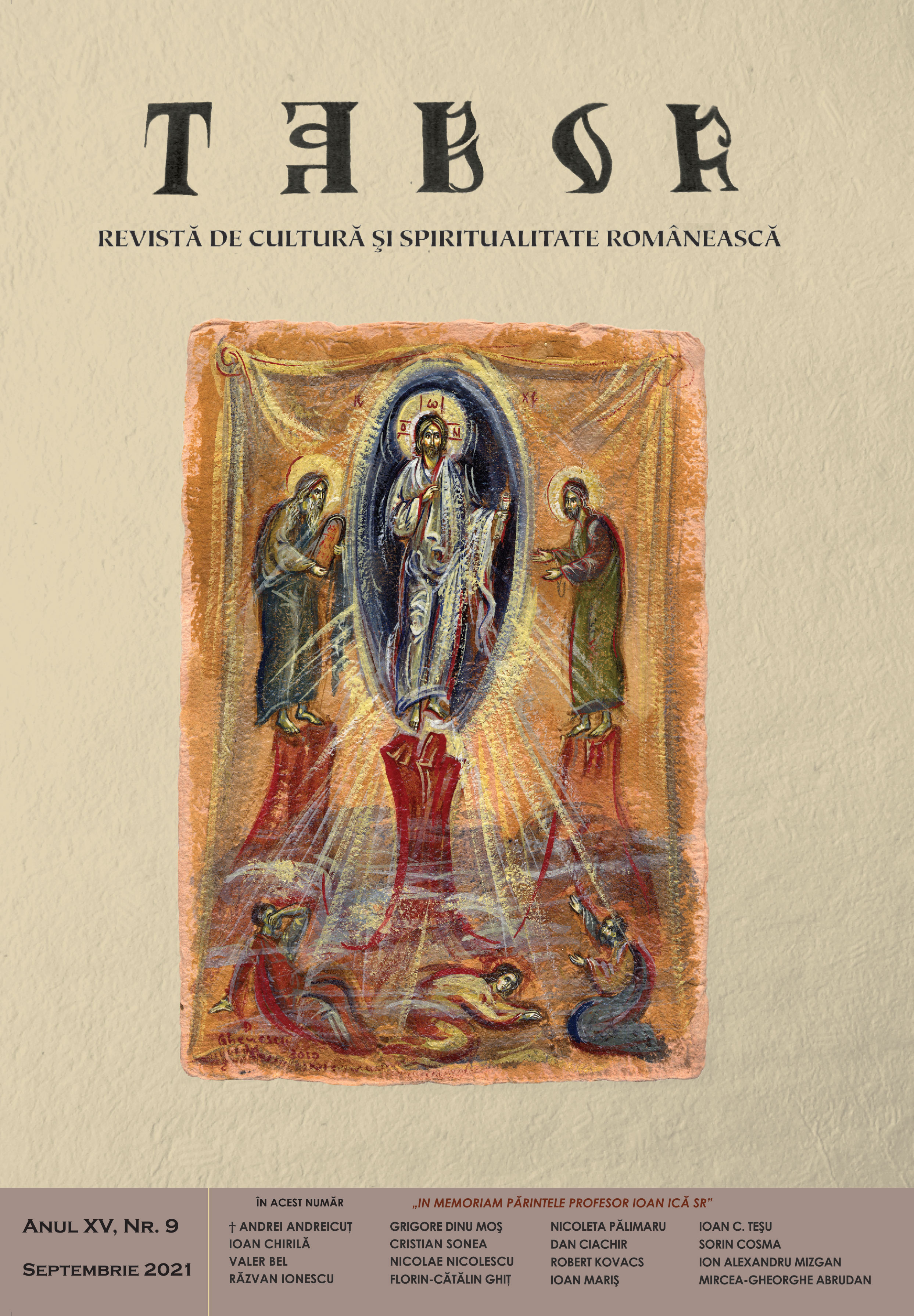This is a color book or magazine cover with an off-white background featuring a central religious painting. The focal point of the painting is a man, presumably Jesus, at the center encircled by a glowing oval, with two robed men to his left and right, each with glowing halos around their heads. Jesus, depicted in a white robe and holding a shaft, is accompanied by followers prostrated and worshiping at his feet. The title at the top reads "Tabor" in large, bold text, followed by "Revisita de Cultura si Spiritualitate Romanesca," indicating Romanian cultural and spiritual heritage. At the bottom left, in a brown band, is black text stating "Anu XV, NR 9, September 2021, in memoriam Parentele Professor Iona Ica, Sr." This caption is followed by a long list of names and additional information about the publication date.